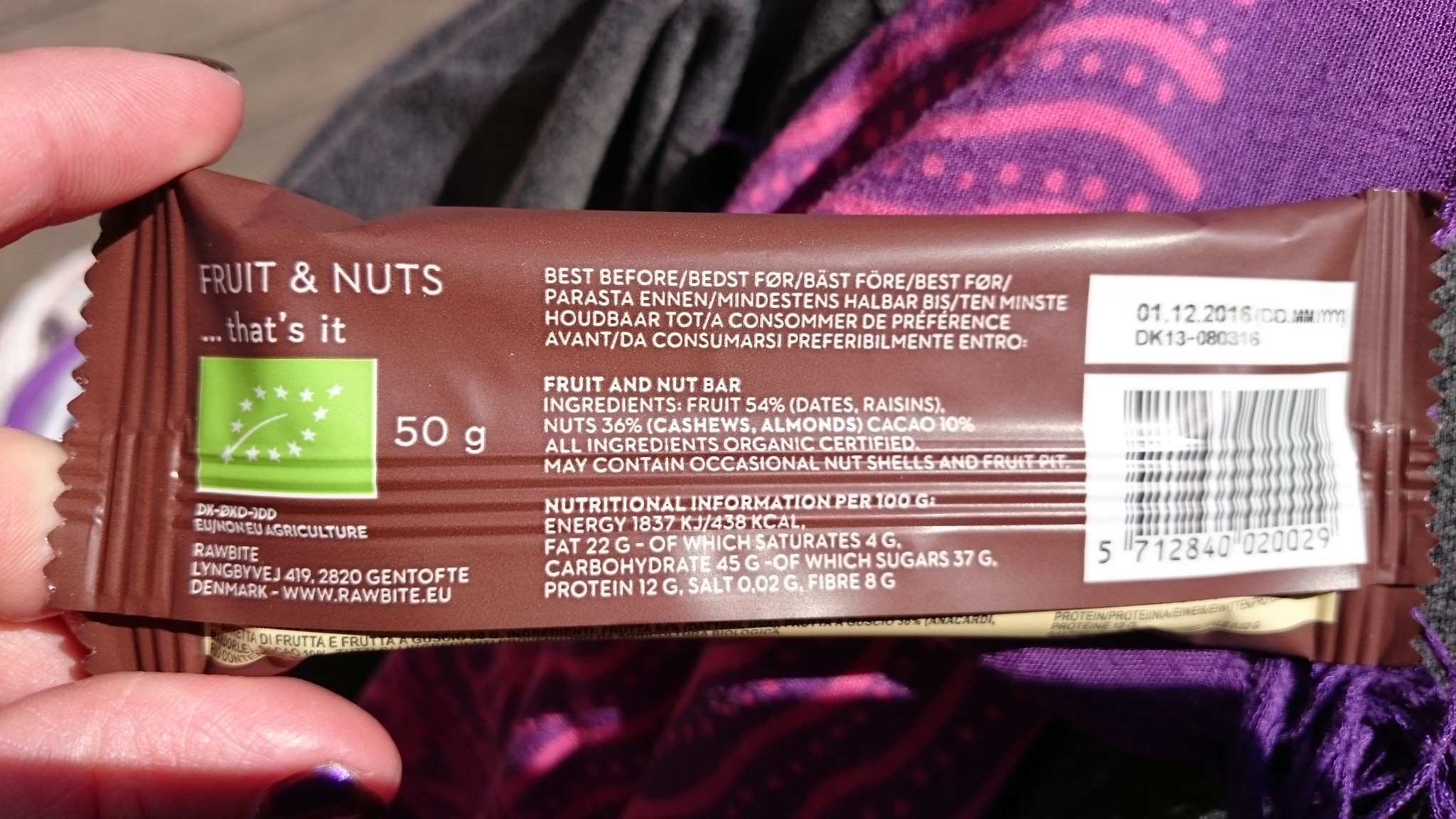In this image, we see the backside of a fruit and nuts bar packaging. The packaging is predominantly brown. At the top left, the design includes the text "Fruit and Anisine" followed by "Nuts" beneath it, and then "…That's it." Directly below this text is a light green shaded square with a starry design around it, resembling a leaf shape, and it contains the text "50g."

To the right of the design, the packaging displays the list of ingredients in multiple languages. The English ingredient list is centrally positioned. Below the ingredients section, there is nutritional information per 100g.

On the right-hand side of the packaging, there is a white label with a barcode directly underneath it, contained within a white square. The bar is being held by two fingers emerging from the left side of the image.

The background under the bar includes a purple blanket with pink designs, a gray blanket to the left, and a gray flooring background in the top left corner of the image.